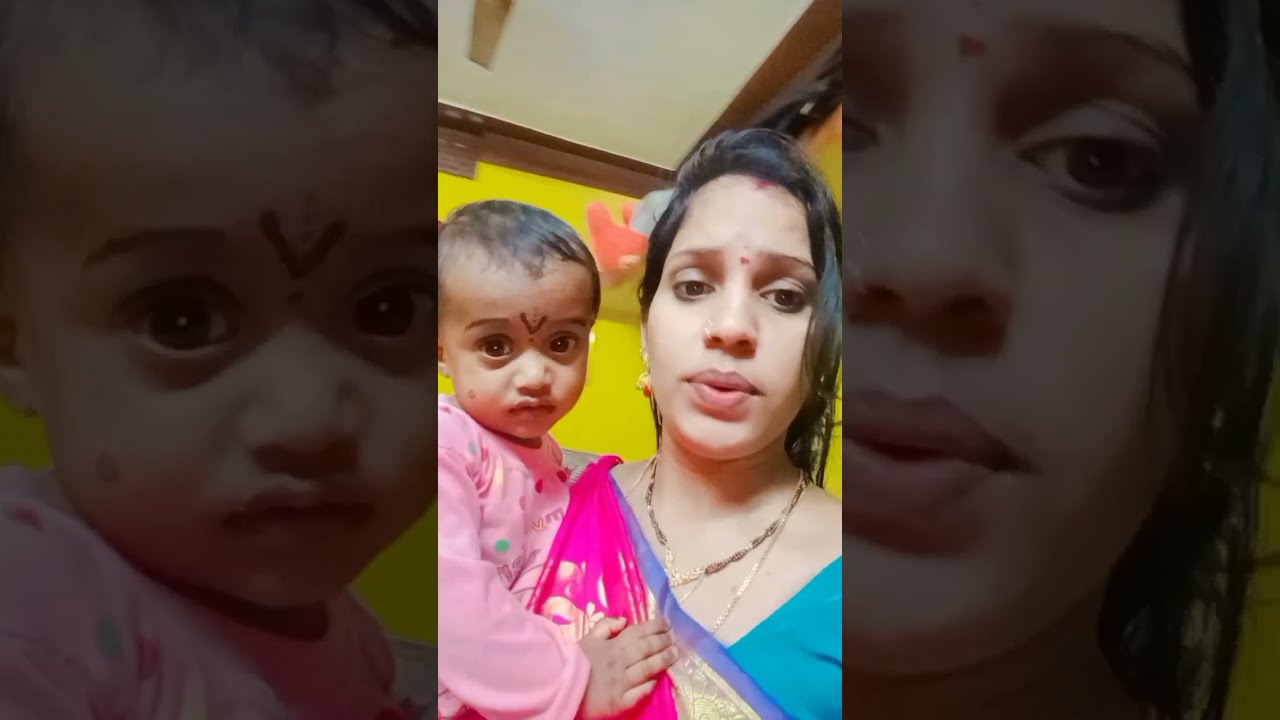In the center of the image, a young woman, likely around 19 or 20, is holding a little girl, who appears to be about 2 or 3 years old. The woman has black hair and wears a sari in shades of pink, blue, and purple. She accessorizes with necklaces and a nose ring and has a light pink dot between her eyes, possibly indicative of being from India. The child, dressed in a pink shirt, has short black hair and features a distinctive V-shaped marking on her lower forehead between her eyebrows. 

The background of the image is a neon yellow wall with indistinct pink elements on it, and the ceiling is light gray. The main colors in the image are tan, pink, and yellow. On the left and right sides of the photo, there are slightly faded and zoomed-in versions of the central image, enhancing the focus on the woman and child. The image seems to be a selfie taken indoors, possibly in a setting reminiscent of a third-world country, and it may have been captured via a mobile app like TikTok or Instagram.